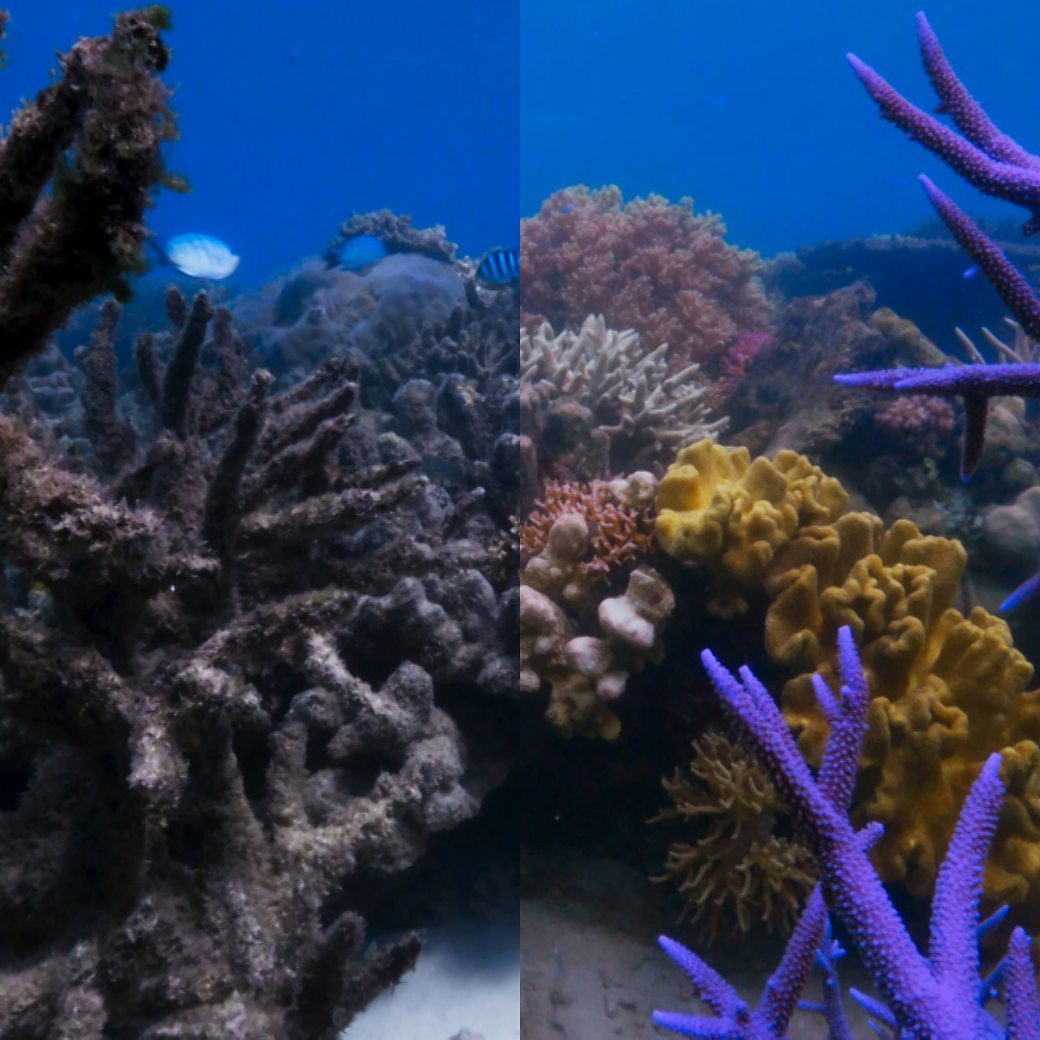This image depicts an underwater scene split into two panels, likely taken either at different times or locations, highlighting a stark contrast between a damaged and a thriving coral reef. On the left side of the image, the coral appears brown, burnt, and unhealthy, with a dark background that includes some fish, possibly angelfish, swimming through. The corals here seem lifeless and bleached out. Conversely, the right side of the image bursts with life and color, featuring vibrant, healthy corals in various hues. Notable details include finger-like purple corals with lighter circles and dots, yellow brain-patterned corals, and whitish coral in the background. The water on this side is a lighter blue, showcasing a range of colors from blue and pink to orange and white, making the contrast with the left side even more striking. The overall scene demonstrates the dramatic difference between a stressed, bleached coral reef and a flourishing, diverse ecosystem.